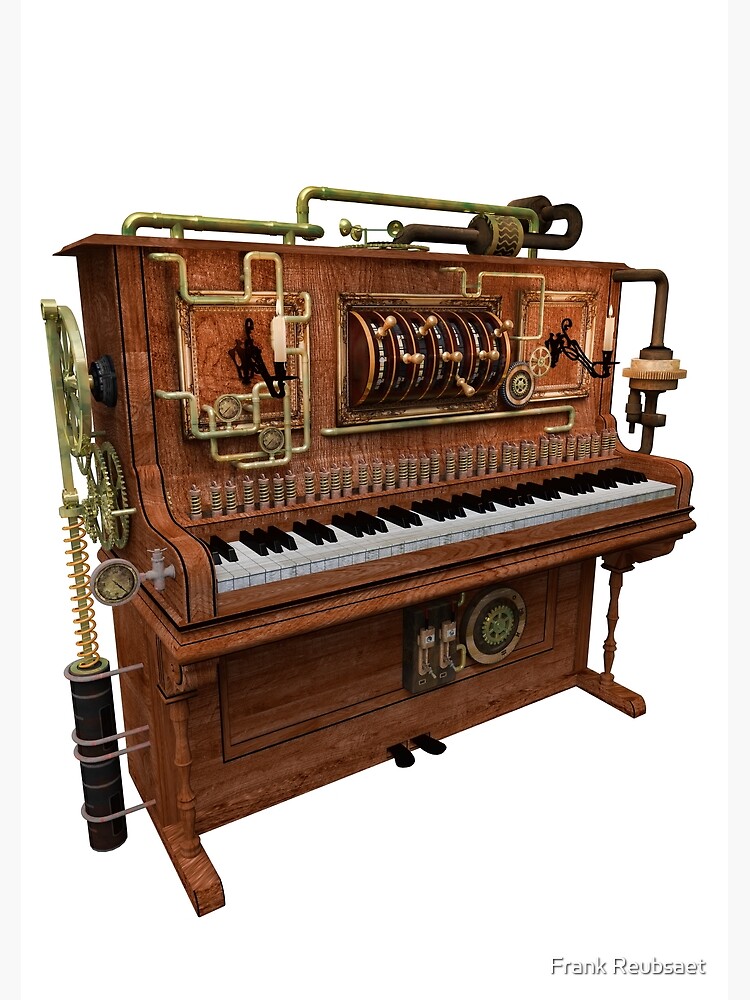The photo depicts an ornately designed piano, featuring a steampunk aesthetic. The piano is primarily made of natural brown wood and showcases a mix of black and white keys, anchored by two foot pedals at the bottom. Above the pedals is a complex contraption resembling a wheel and a box. The left side of the keyboard has a clock hanging off it. The piano's top and sides are adorned with cranks, spindles, handles, and various doodads, giving it a slot machine-like appearance at some points. This intricate assembly also includes numerous levers, specifically seven centered on the top front, accompanied by pipes, some of brass color, and other metallic features. There are gears and other mechanisms throughout, contributing to its elaborate design. Additionally, there are candles on both the left and right sides of the piano. The background is white, and in the bottom right corner, there's a watermark with the name "Frank Rupset."